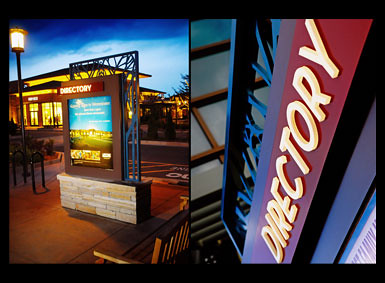The image is a square with a thicker black border on the top and bottom and a thinner black border on the sides. It appears to be a screenshot from a video game or possibly digital art. The background showcases a dark blue sky that transitions into a lighter blue, suggesting it's evening. There is a small patch of green, some visible buildings with lights on, and an outdoor seating area with a table and chairs, although details are somewhat indistinct. A lit streetlight indicates the time of day.

The central focus is an urban outdoor scene characterized by surreal, bright colors. Prominently, there is a directory sign, mounted on a stone base, positioned beside a bus stop. This black sign features the word "Directory" in white letters. To the right, another larger, diagonal directory sign appears, with white bubble font against a black bar on a maroon-colored wooden background, framed by hot blue metal. Additionally, there are metal rails presumably for securing bicycles and a bench nearby, enhancing the urban environment ambiance. The image might be split, showing a close-up of the directory sign on one side, adding to the layered detail of the scene.